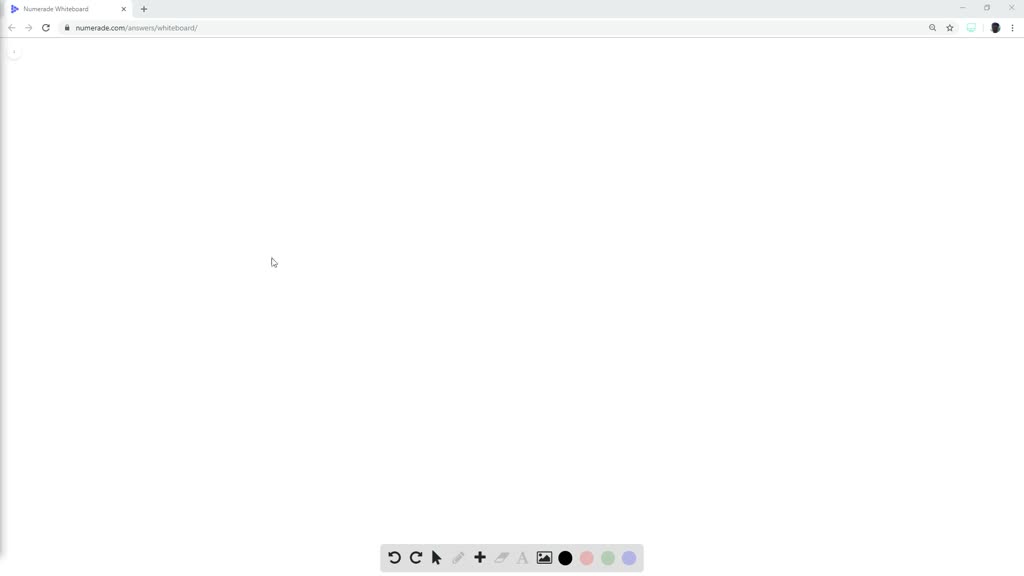The image is a screenshot of a computer interface, specifically a web-based application. The screenshot depicts a rectangular window oriented horizontally, mimicking the shape of a standard computer screen. This window has a gray border only along the top and left sides, leaving the bottom and right sides against a plain white background.

On the left side of the window, a vertical gray line extends downward, while a horizontal gray bar occupies the top portion. The central area of the screen is predominantly white. Positioned at the very top left corner, the text "Numeraid Whiteboard" is visible within a small white area, followed by the website address "numeraid.com/answers/whiteboard." To the right of this text, standard window control icons are present: a minus sign for minimizing, a square for maximizing/restoring, and an 'X' for closing.

At the bottom center of the image, there is a long, slender gray rectangle that serves as a toolbar. This toolbar contains various symbols, including:
- A circular arrow pointing left (possibly representing an undo function)
- A circular arrow pointing right (possibly representing a redo function)
- A black arrow pointing Northwest
- A crayon icon (likely for drawing)
- A black plus sign
- An icon resembling the letter "A"
- An image icon

Additionally, the toolbar features four colored dots: black, pink, green, and purple, which might be used for selecting colors or tools.